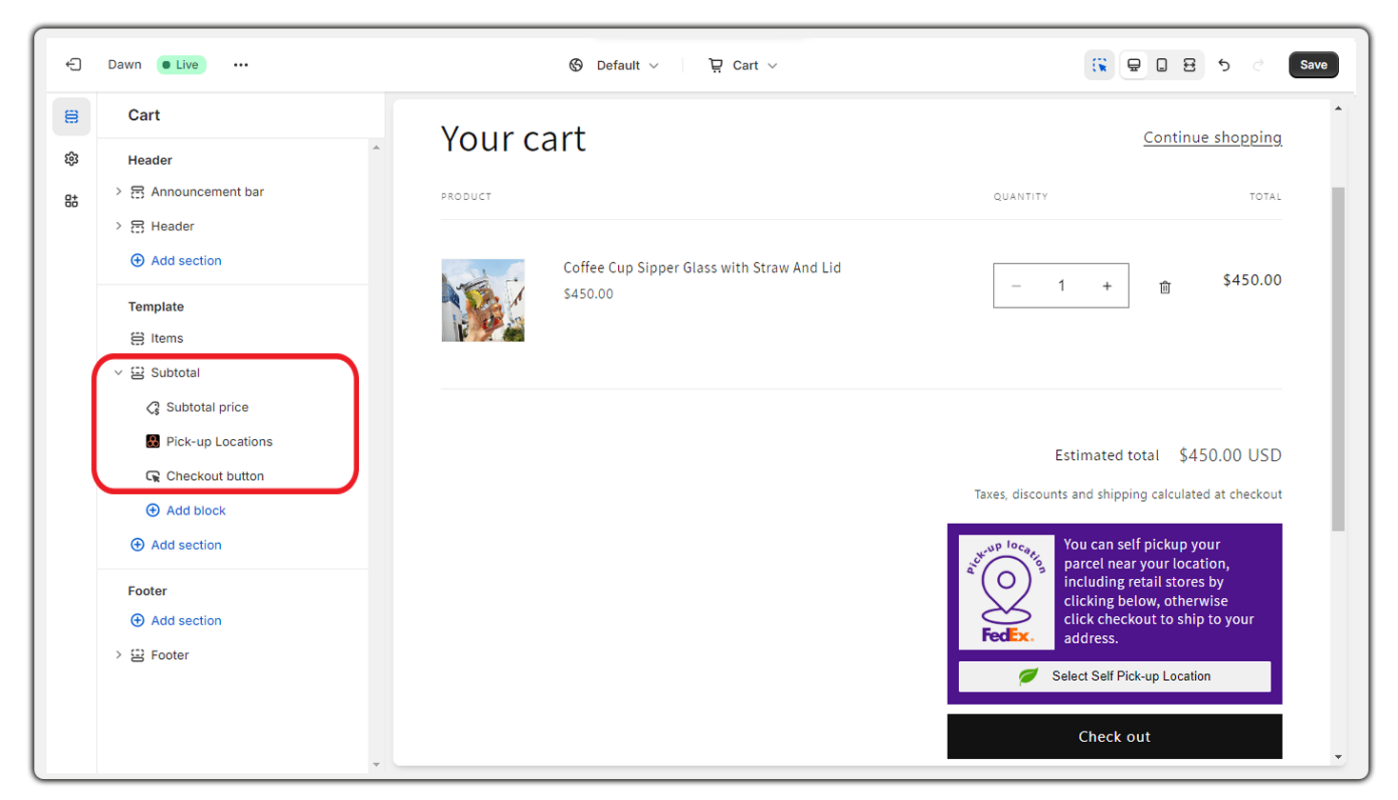Here is a detailed and cleaned-up caption for the image described:

---

The image showcases an online shopping app's website builder interface against a white background. Starting from the top left, there is a "Sign Out" button followed by the word "Dawn." Next to it is a green "Live" button, accompanied by a three-dots menu icon for additional options. At the center of the top bar, the word “Default” is displayed, suggesting a default or language selection. The second option on this bar is a cart icon.

On the far right of this top bar, there are several small icons: a cursor, a desktop monitor, a smartphone, and an icon resembling a split-screen view. Additionally, there are backward and forward arrow icons, followed by a save button.

On the left side of the screen, there's a prominent vertical menu, beginning with a "Cart" section at the very top. Below it, the "Header" section includes options for an announcement bar, a header, and an "Add Section" button in blue. The next primary section is "Template," featuring options for items, subtotal, pickup locations, and a checkout button, all boxed in red. Under this, there are "Add Block" and "Add Section" buttons, both in blue. The final section is "Footer" which has an "Add Section" button and a "Footer" option.

In the main content area of the website builder, the top left reads "Your Cart," with a "Continue Shopping" link to its right. Beneath is a section displaying an image of a coffee sipper cup with a straw and lid, priced at $4.50. Next to it is a small box to adjust the quantity, currently showing "1," accompanied by a total return value. 

At the lower right corner, the estimated total is shown as $4.50 USD, with a note below that taxes, discounts, and shipping will be calculated at checkout. The section also includes a purple box with a FedEx logo, stating, "You can self-pick up your parcel near your location, including retail stores by clicking below. Otherwise, click checkout to ship to your address." 

Below this message, there is a prominent black "Checkout" button.

---